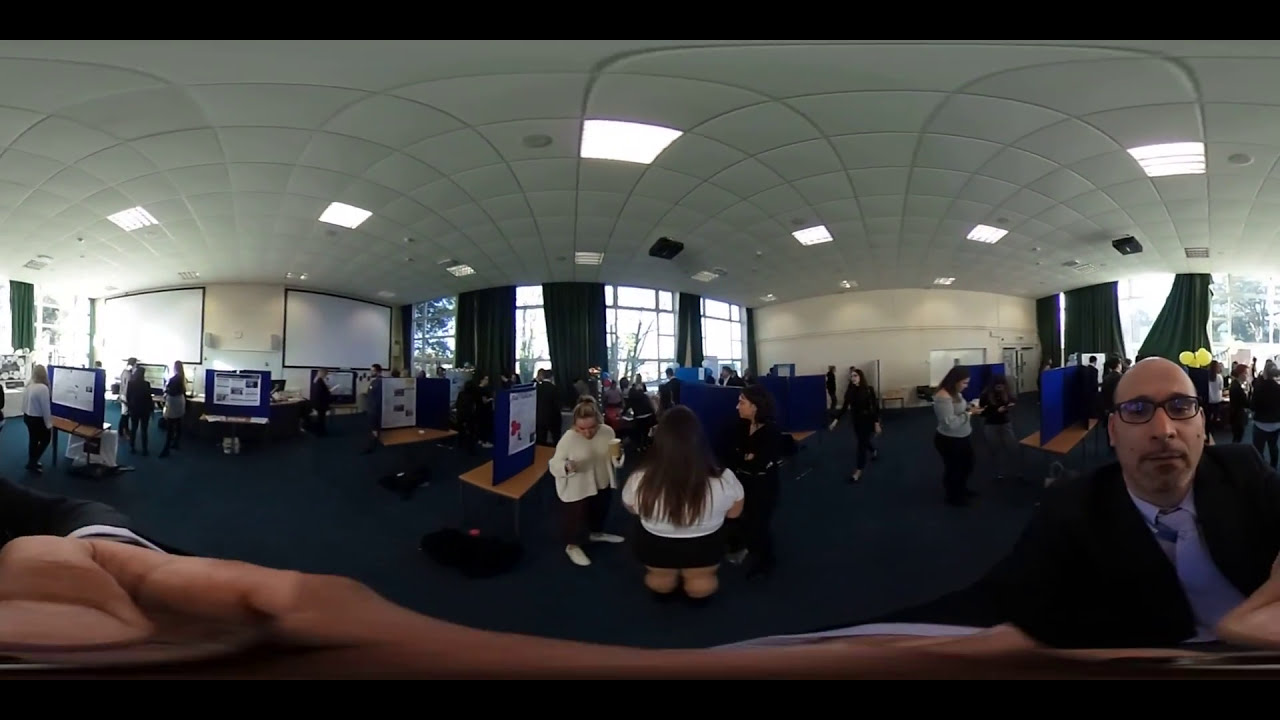This image captures a panoramic view of a convention or expo with a slight fish-eye distortion. In the foreground to the right, there is a bald white man with glasses wearing a blue shirt under a black jacket, and he also has some stubble. His hand appears slightly distorted at the bottom of the image, as if he is touching or adjusting the camera. To the left of the foreground, a woman with long black hair, a white shirt, and a black skirt is seen from behind. Nearby, another woman is visible, wearing a white sweater with black pants and possibly tennis shoes, with her hair pulled back. The room features several displays and round tables with poster boards, indicating a bustling environment where people, including multiple women, are walking around and examining the presentations. The background shows large windows with black drapes, along with white walls, a white ceiling with fluorescent lights, and blue carpeting. The setup and atmosphere suggest that this is a presentation hall or science fair where attendees engage in discussions and display their work.